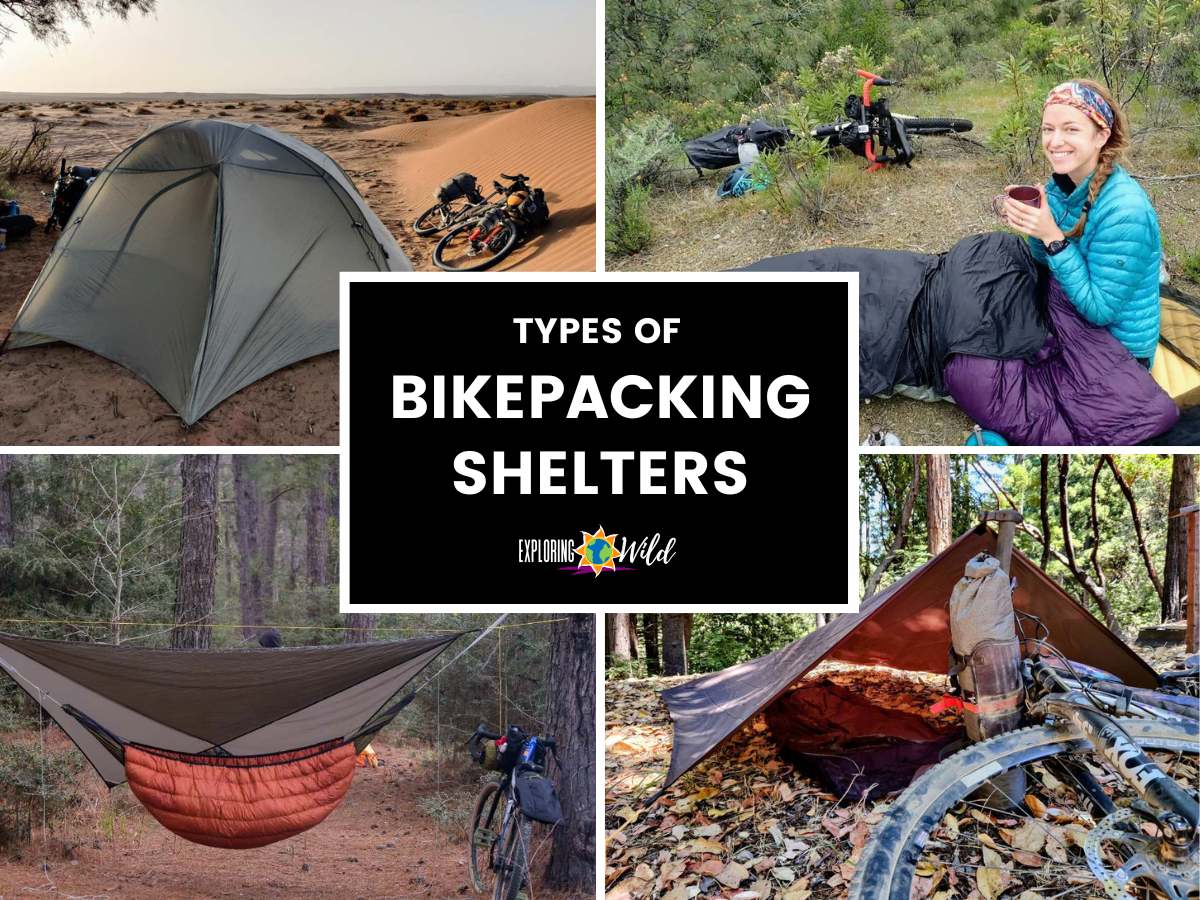The image is a collage of four distinct outdoor scenes, each illustrating a different type of bikepacking shelter, with a central black text box containing the title "TYPES OF BIKEPACKING SHELTERS" in white, all-caps text, and the tagline, "Explore Wild." 

The top left photo depicts a gray tent pitched at the edge of a desert sand dune with a bicycle resting nearby on the sandy hill, illuminated by sunlight. The top right photo shows a young girl in a black and purple sleeping bag. She is sitting up, holding a red cup, and smiling at the camera. She's dressed in a blue winter jacket and a headscarf, with a bike lying on the grass behind her in a lush, green forested setting. 

In the bottom left image, a red hammock is suspended between two trees in a forest, with a bike leaning against one of the trees nearby. Lastly, the bottom right photo presents a makeshift tent fashioned from a tarp set up in a forested area, bathed in sunlight, with a bicycle lying on the forest floor outside the tent. 

Together, these images vividly showcase various bikepacking shelters in scenic outdoor environments.